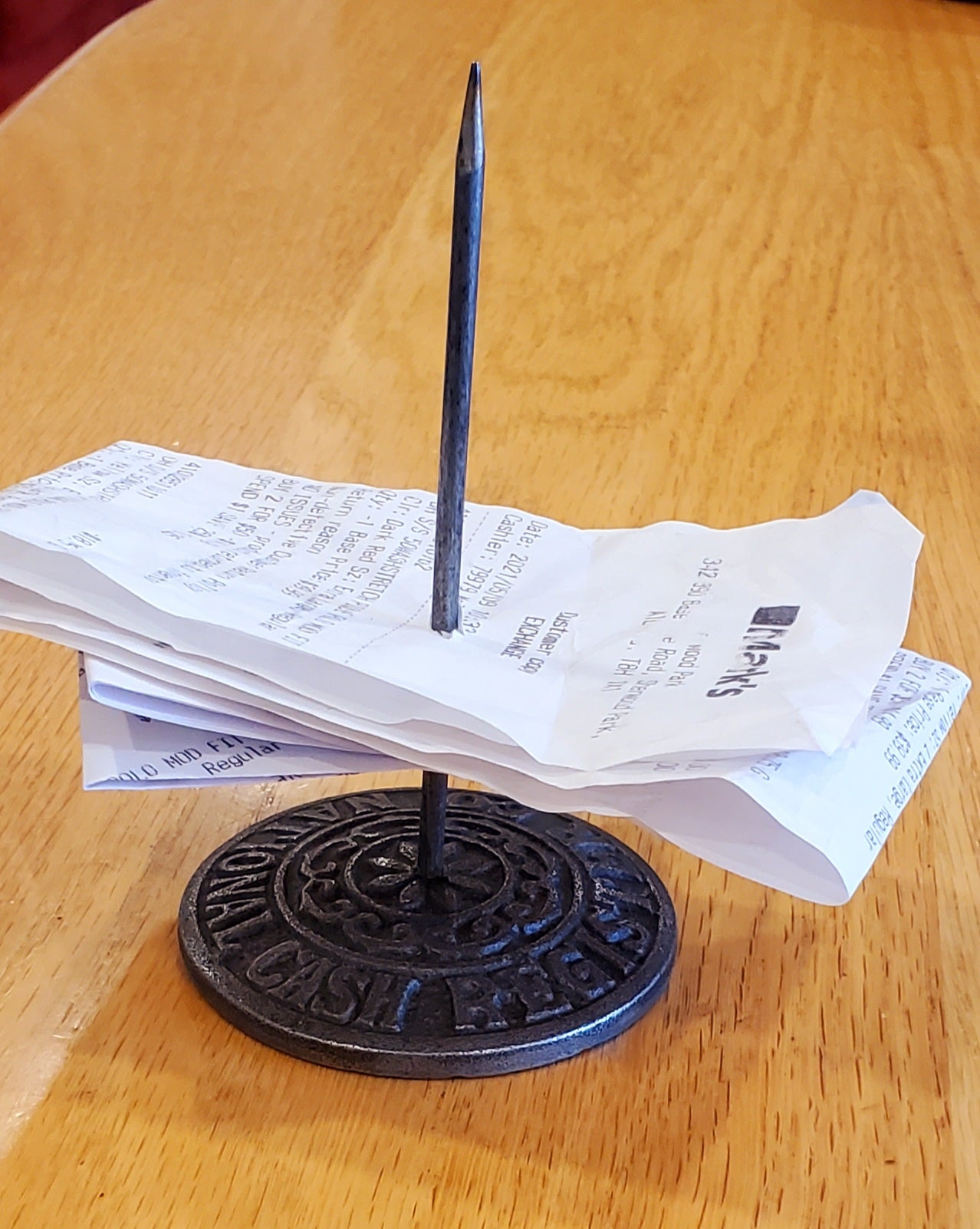This is a close-up photograph showcasing a vintage receipt holder prominently displaying several receipts. The holder features a cylindrical black base with intricate embroidery encircling it, reading "National Cash Register," and a floral design at its center. From this base emerges a long, thin metal spike, sharp and seemingly designed for easy puncturing of receipts. The spike supports an array of receipts from different companies, with one identifiable slip from "Marks," dated June 9th, 2021, displaying partial address details and the cashier's number. The holder rests on a light brown wooden table with darker stains in the top right corner, and to the left, the image reveals a maroon-colored wooden floor. The overall setting is well-lit, providing clarity to the rustic and somewhat hazardous nature of the receipt spike.